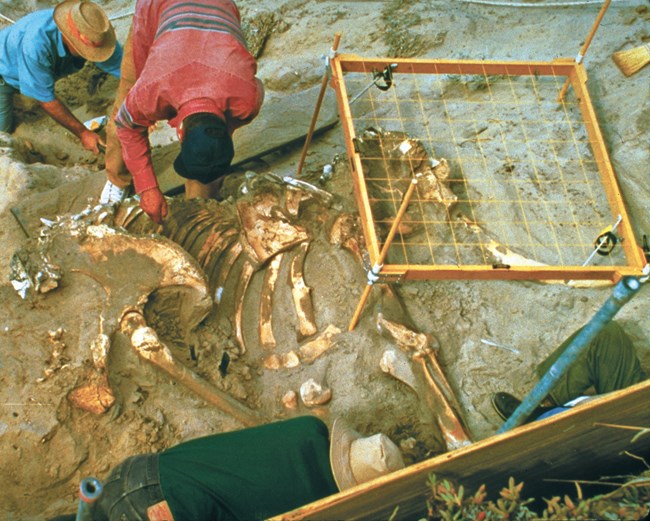In this bird's-eye view of an outdoor archaeological dig, four archaeologists diligently work on excavating what appears to be the bones of a large, possibly extinct animal, potentially a dinosaur. Two men are prominently visible in the top left of the image; one wears a red, long-sleeved shirt with stripes at the elbow and a black hat, while the other, further back, dons a blue shirt and a white sombrero with a band. To their right, there is a wooden sifter with a grid top, positioned above the bones to filter out rocks and dirt. In the foreground, a third man bends over in a green shirt and a white hat, closely examining the ground. The feet of a fourth archaeologist can just be seen in the lower-left corner of the image, suggesting their focus on the excavation as well. The surrounding area appears rough and concrete-like, with a partial wall visible near the bottom right, enhancing the industrious atmosphere of the dig site.